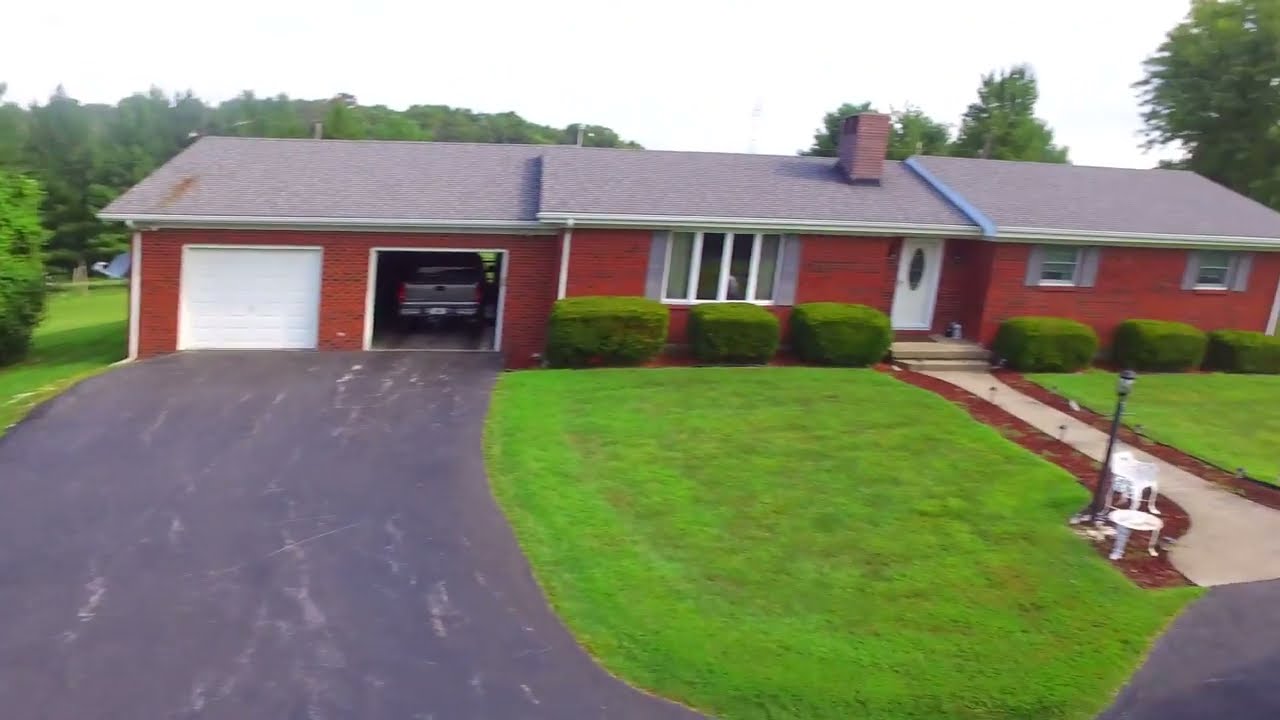The photograph depicts a single-story red brick suburban house with a grey, conical slanting roof. On the left side, there is an open two-door garage where a grey pickup truck is parked. The garage door is white, and a blacktop driveway leads to it. To the right of the house, the main entrance features a white door with a vertically oriented thin oval glass window. A cement walkway, bordered by reddish wood chips, extends from the front door towards the street, intersecting with a manicured green lawn.

In front of the house, there are two large rectangular hedges alongside the white-framed windows. Additional smaller windows are present across the facade. The center of the lawn hosts a small white chair and table setup, right next to the walkway. This area also connects to a green path leading to the garage. The house sports a chimney above the entrance area.

On the right side of the main house is another structure that appears to be an extension, similar in design but lacking a chimney. The entire property is adorned with green trees in the background, and the sky appears overcast or white.